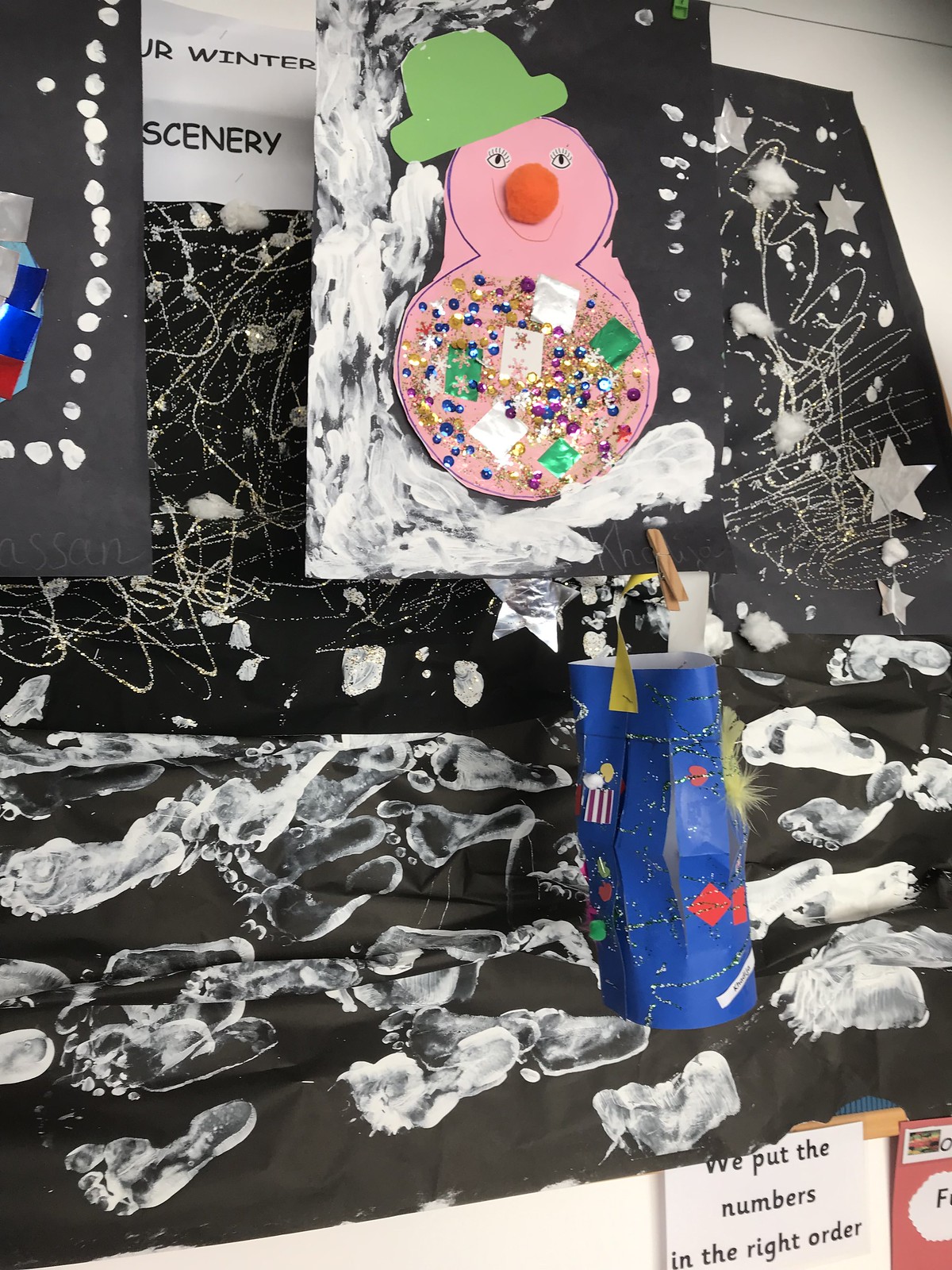The image depicts a vibrant bulletin board, likely inside a classroom, showcasing children's winter-themed art projects. Dominating the display is a creatively crafted pink snowman made from construction paper, adorned with a green hat and a prominent orange nose. The snowman's body is festooned with an array of blue, gold, and purple sequins, adding a shimmering effect. The backdrop of the bulletin board is black, also constructed from construction paper, and is speckled with white paint to simulate falling snow.

To the right of the snowman, there's a piece of paper with the inscription "Our Winter Scenery." Beneath this title, more of the black background is visible, decorated with white footprints, suggesting the playful involvement of the children in the project. A single blue package, possibly a Christmas present, is situated centrally in a festive bag. At the very bottom of the board, a white piece of paper with neatly ordered black numbers declares, "We put the numbers in the right order." The scene is a delightful blend of color, texture, and creativity, encapsulating a charming winter wonderland as imagined and crafted by children.